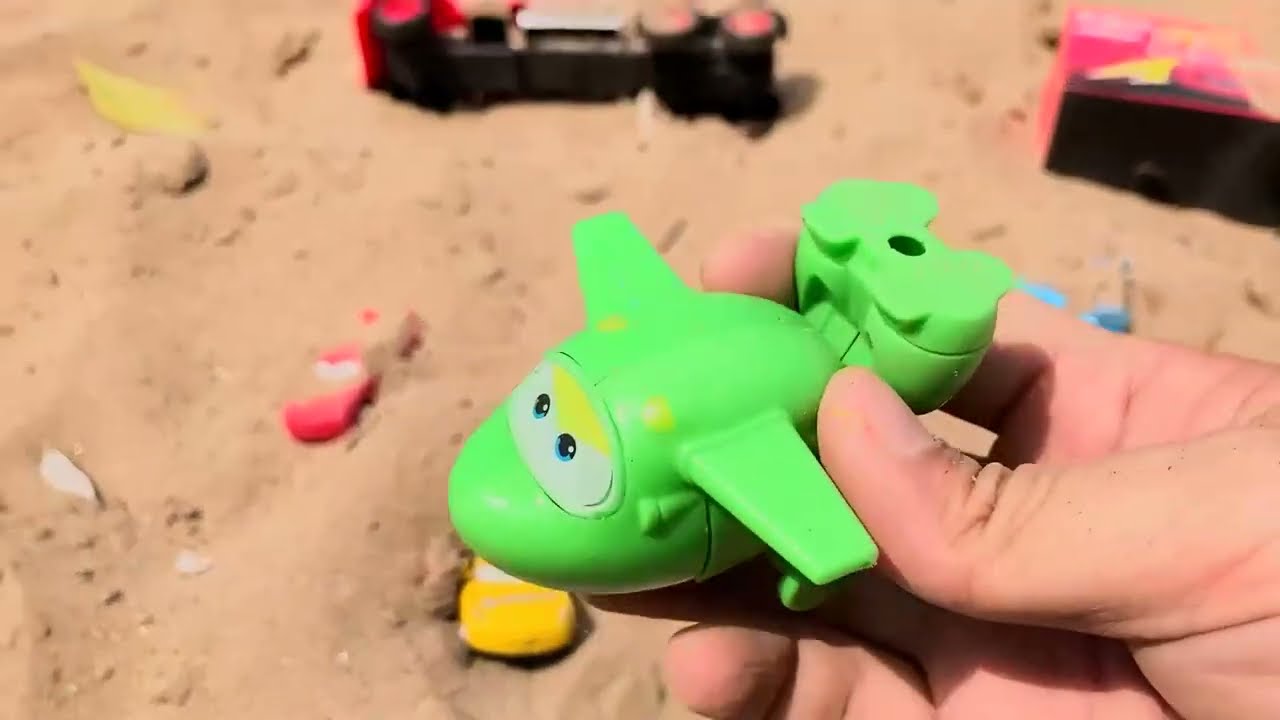The image captures a detailed scene of a sandy area filled with various children's toys. In the bottom right corner, a person's hand, with light-colored Caucasian skin and very short clipped fingernails, extends into the frame, holding a small, light green toy airplane. The toy airplane features a white windshield decal with blue and black eyes, resembling a character from the Disney movie "Cars." A yellow strip runs just above the eyes, and there are yellow dots on top of the airplane. Its wings are outstretched, with one touching the person's thumb.

In the background, a landscape of scattered toys in the sand is visible. To the left of the airplane, there's a red toy truck partially buried in the dirt, which looks like Lightning McQueen from "Cars." Above the airplane, a black structure with white circles can be seen, alongside another black structure with square pink parts in the top right corner. There are other partially obscured toys, including a yellow buried car and a blue object in the sand, which might be a scoop. The environment suggests either a sandbox or a beach, with clumps of brown sand scattered throughout, and no text present in the image.